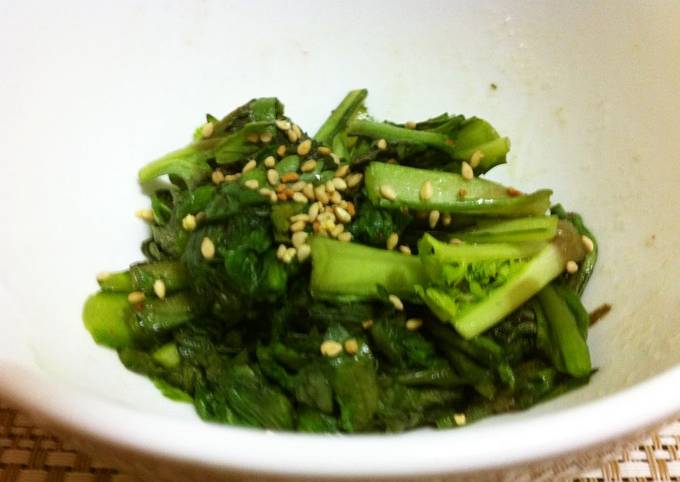This is a close-up, albeit grainy and slightly blurry, photograph of a small quantity of oriental-style food presented in a white ceramic bowl. The bowl is partially visible, primarily along the lower left-to-right part of the image, and appears to be larger than necessary for the portion size. The food inside consists of green vegetables that resemble a hybrid between broccoli and celery, with floret-like tops but stems more akin to celery. The vegetables seem to be either steamed or sautéed, giving them a slightly mushy texture with a light, oily sauce. The dish is garnished unevenly with tan, teardrop-shaped seeds, which appear to be toasted sesame seeds. The bowl is set upon a woven wicker surface or placemat, further highlighting its oriental presentation.